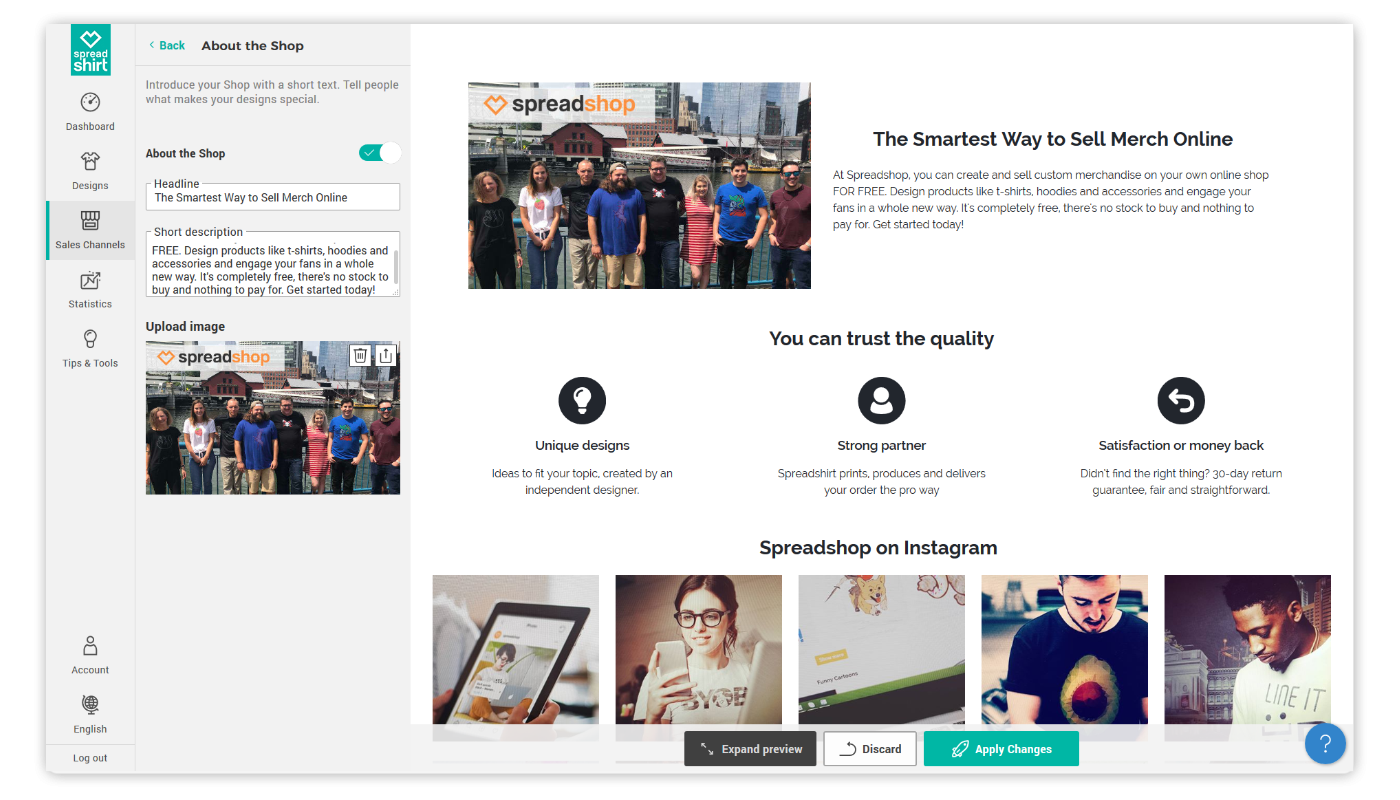A detailed screenshot of a webpage from Spreadshirt displaying information about selling merchandise. The left sidebar, featuring a light gray background at the top, lists various navigation categories. At the top of the sidebar, within a teal blue background, is the Spreadshirt logo. The categories below are: 

1. **Dashboard** with a speedometer icon.
2. **Designs** with a t-shirt icon.
3. **Sales Channels** with a kiosk icon (currently selected, distinguished by a slightly darker gray background and a teal bar on the left).
4. **Statistics** with a chart icon.
5. **Tips and Tools** with a light blue icon.
6. **Account** with a person icon.
7. **English** with a globe icon.
8. **Logout** at the very bottom.

Adjacent to the Sales Channels selection is a column with a light gray background. At the top of this column, "Back" is written in blue text beside a left-pointing arrow. Below this, it reads "About the shop," followed by instructions: "Introduce your shop with a short text. Tell people what makes your design special." 

Continuing further down the page, under another "About the shop" heading, there is a blue toggle switch in the teal position with a checkmark, indicating it is enabled. Beneath the switch, it says "Headline" followed by a text entry box that reads, "The smartest way to sell merch online."

Following this, under the "Short description" heading, the text entry box contains: "Free. Design products like t-shirts, hoodies, and accessories, and engage your fans in a whole new way. It's completely free. There's no stock to buy and nothing to pay for. Get started today."

At the bottom, under "Upload image," there is a photograph of several people standing in a line in an urban setting. In the top left corner of the photograph is the Spreadshop logo, with "Spread" in black text and "shop" in orange. To the right of the image, there are icons for a trash bin and an upload button.